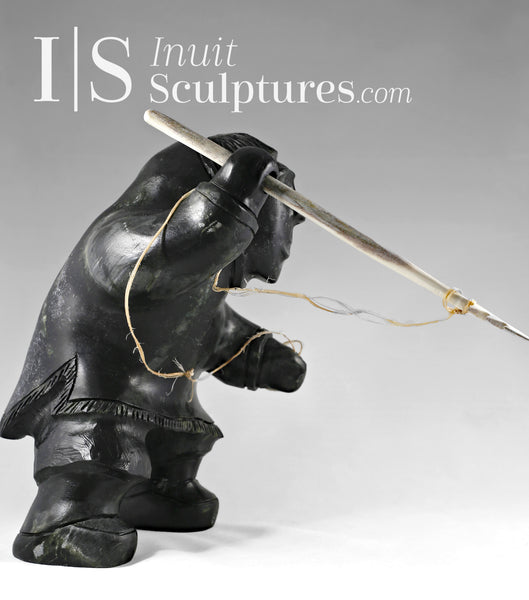The image displays a digital photograph of an intricately crafted Inuit sculpture prominently featuring an Eskimo figure. Positioned in the center is a strikingly black sculpture of a hulking, human-like figure. The Eskimo is garbed in a traditional jacket and trousers, portrayed with a spear in its right hand, with a string connected to the spear also attaching it to the figure’s left hand. The spear is depicted as having a wooden shaft with a pointed, metallic tip. The background of the image is a muted gray, highlighting the dark figure. Additional details in the image include textual elements reading "InuitSculptures.com" at the top left, with "dot com" in an italicized serif font. The overall color scheme is dominated by shades of black, gray, with subtle infusions of white, brown, and silver, lending the piece a somber yet striking visual narrative.